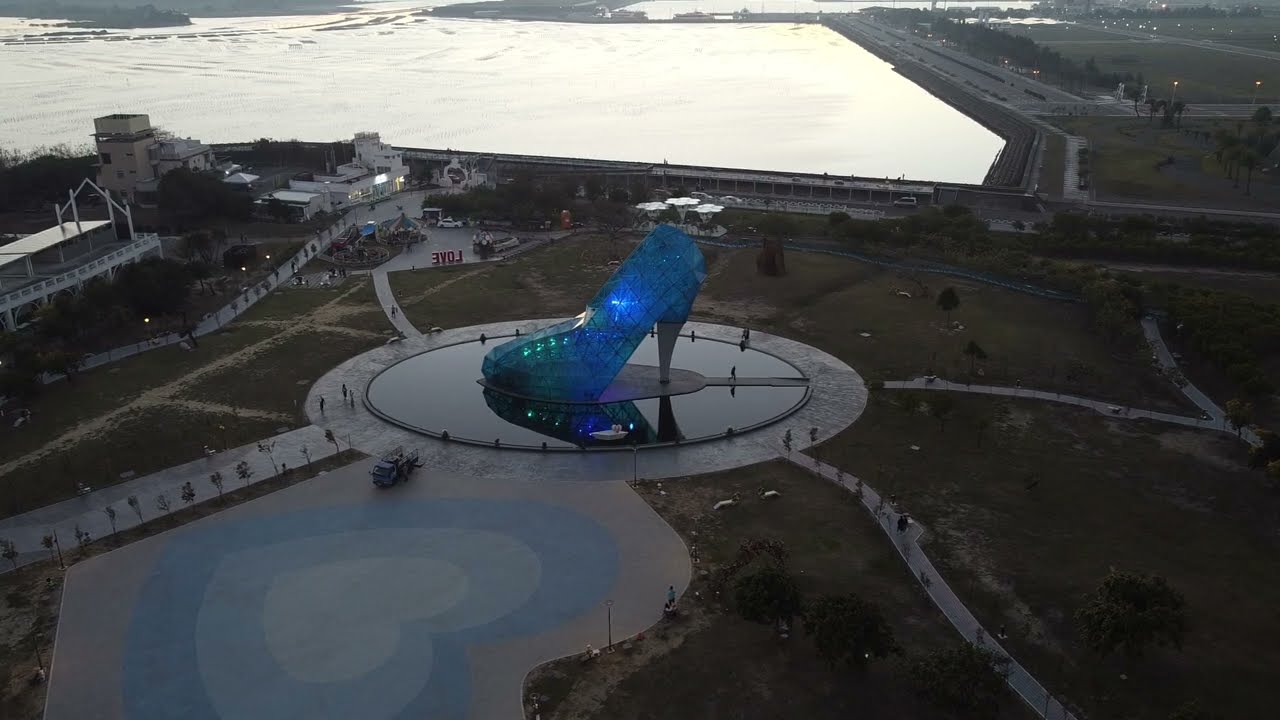The image depicts a well-maintained amusement park, viewed from an aerial perspective. At the center of the scene, perched on a stone circular structure surrounded by water, is an enormous blue glass slipper, significantly larger than the surrounding buildings. Adjacent to this monumental slipper is a large blue heart integrated into the ground, reminiscent of a city square, arranged in concentric layers of varying shades of blue. Well-trodden paths radiate from the circular centerpiece, populated by visitors strolling through the park. In the upper left of the image, buildings suggest a leisure area, possibly featuring carnival rides. The background includes a neatly edged body of water bordered by more paths and trees. Scattered throughout the park are signs bearing the word "Love," but there is no further indication of the park's name or location.